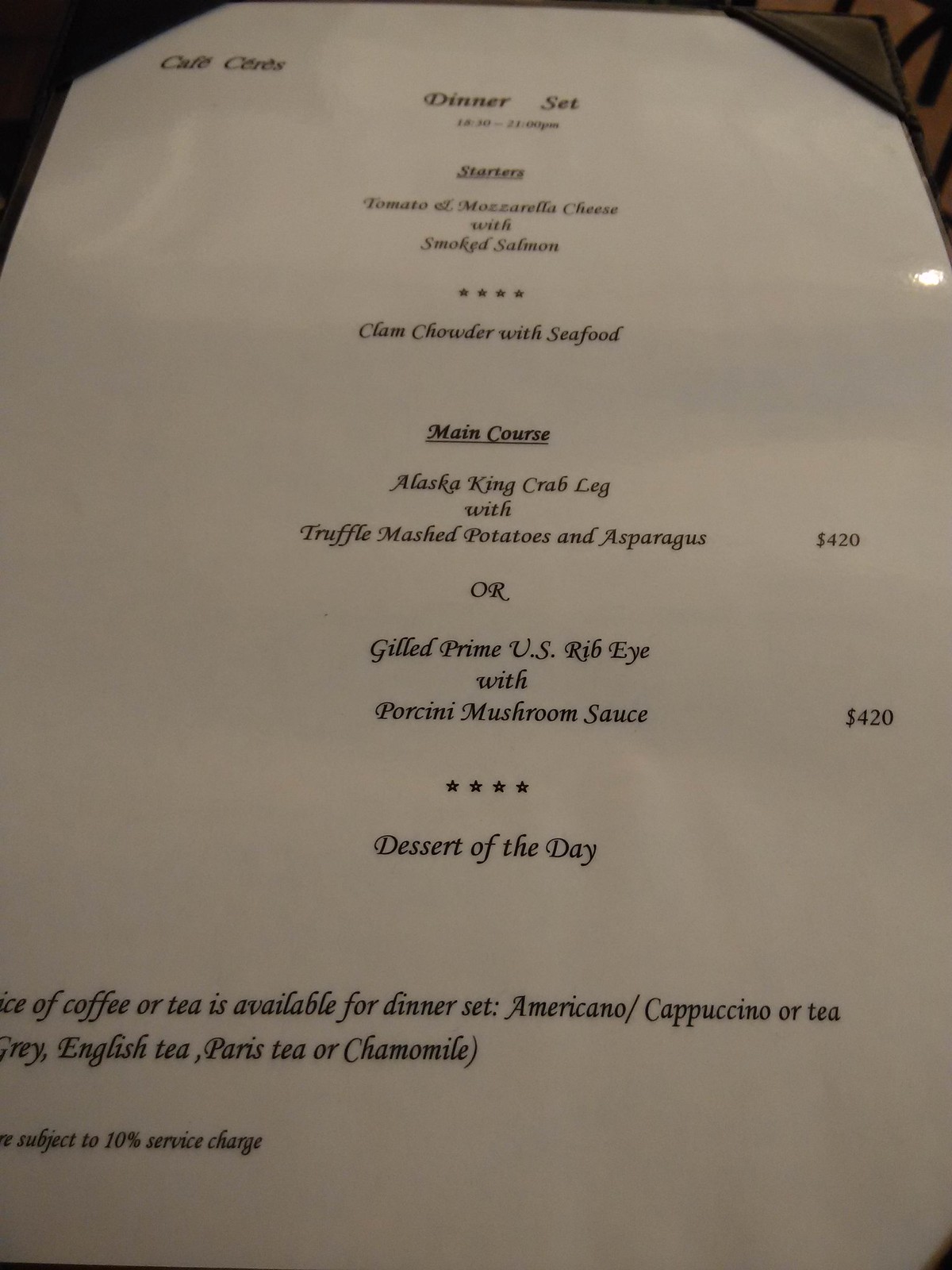This image features a somewhat cropped view of a menu encased in a hardback cover with leather corners that secure the paper in place. The menu, from a restaurant named Café Ceres (or possibly Café Certes), details the dinner set offered from 18:30 to 21:00. The starters listed include "Tomato Mozzarella Cheese with Smoked Salmon," which is visually segmented by a row of four stars from the "Clam Chowder with Seafood." For the main course, there is "Alaska King Crab with Truffle Mashed Potatoes and Asparagus" priced at $420, followed by "Grilled Prime US Ribeye with Porcini Mushroom Sauce" priced at $422. Another row of four stars separates these items from the "Dessert of the Day." At the bottom of the page, though partially cut off, it can be seen that the dinner set includes a beverage choice, offering options such as "Americano/Cappuccino or Tea," with tea selections including "Earl Grey, English Tea, Paris Tea, or Chamomile." Finally, in small print at the bottom, the menu notes that prices are subject to a 10% service charge.